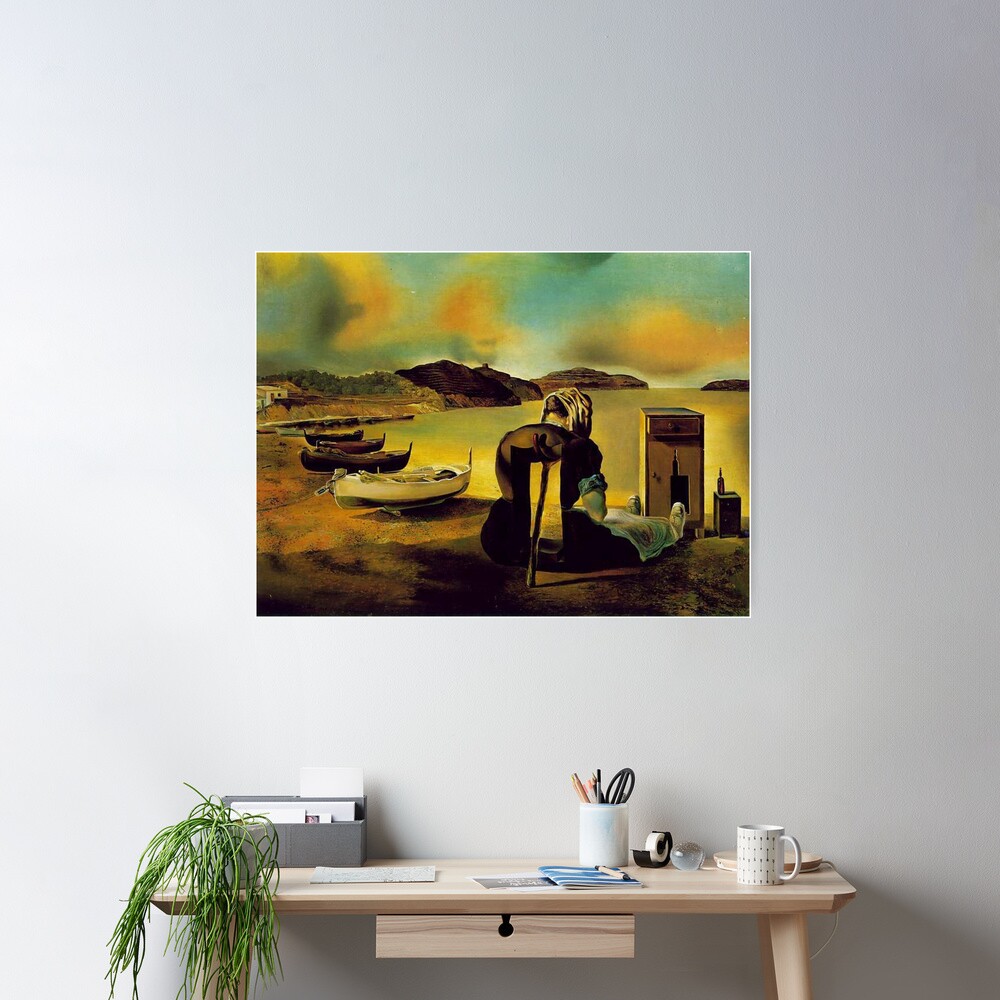This photograph features an image of a room rooted in modern minimalism, dominated by a sleek, pale-wood desk pressed against a stark, white wall. The desk is sophisticated in its clean lines and minimalist design, with a functional pull-out shelf hiding underneath. The surface of the desk hosts a variety of items, meticulously arranged: a white desk lamp sits at the far right, followed by a white coffee mug, a glass paperweight, and a tape dispenser. Adjacent to these, a white container houses scissors and pens, while towards the left, a gray tray holds papers and a small green plant in a white pot adds a touch of nature. The legs of the desk are out of sight, contributing to the airy and uncluttered ambiance of the scene.

Dominating the visual focus of the room, an abstract painting is centrally mounted on the pristine white wall above the desk. The painting is a vivid burst of color in an otherwise monochrome setting, featuring a landscape with blue skies streaked with orange clouds and an orangey-red mountainous backdrop. The striking depiction includes three boats moored by a body of water, with detailed elements in the foreground resembling a bed, a person lying with visible feet, and a peculiar headboard morphing into human-like arms and head, evoking influences of Salvador Dalí. The dream-like, surreal quality of the artwork stands in stark contrast to the room's minimalist, modernist setting, making it the captivating centerpiece of the photograph.